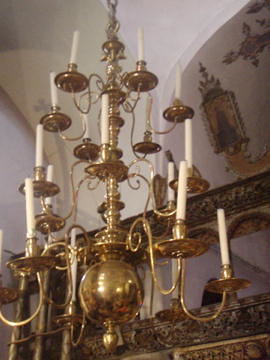The image depicts a small, low-quality, vertical rectangular photograph of an ornate gold chandelier, seemingly cropped and compressed. This chandelier, hanging from a white vaulted ceiling (partly visible in the background), is structured in a cone-like fashion with four distinct, graduated layers, resembling a pyramid. It features intricate design elements, including curving loops extending from its base to support candleholders, each adorned with long, thin, white candlesticks. These candlesticks, set atop dishes-like tiers at various heights, add to the chandelier's elegant and historic aesthetic. In the background, arches and possibly other ornate elements can be faintly observed, contributing to the sophisticated ambiance of the scene.